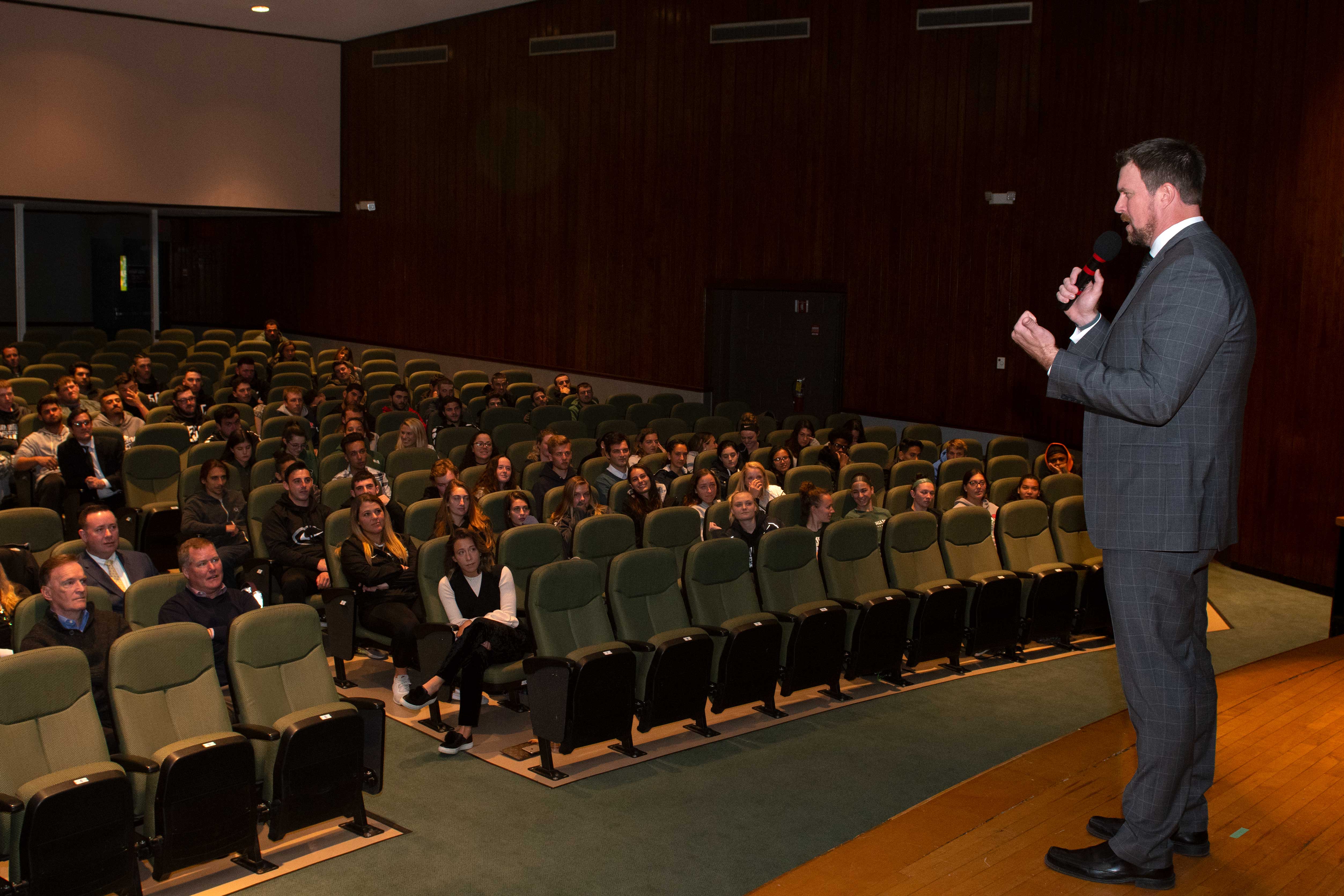In a dimly lit auditorium, a Caucasian man in his 30s or 40s, dressed in a full gray suit and black shoes, stands on a wooden stage holding a black microphone with red strips in his right hand. He has short brown hair, a beard, and a mustache. Positioned on the right-hand side of the image, he is facing slightly left, towards the nine o'clock position. The room features a mixture of dark red and white walls, with the white wall visible in the upper left-hand corner. The auditorium is filled with rows of olive green movie theater-style seats. Scattered throughout these seats are men and women of various ages, filling about a quarter to a third of the available seating. The audience is intently listening to the man, who appears to be delivering a speech or presentation at a speaking convention or similar event.